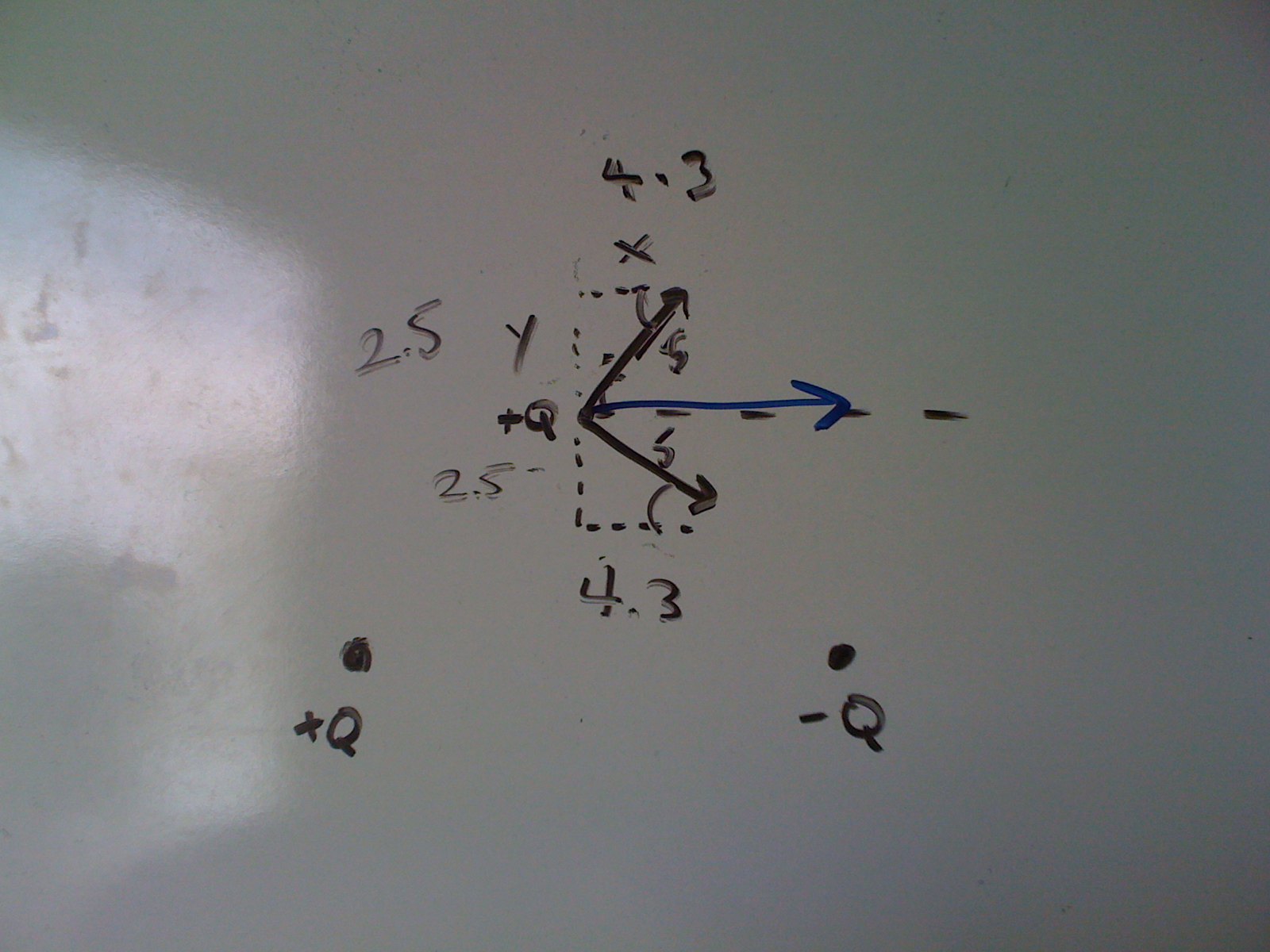This close-up photograph captures a slightly dimly lit whiteboard displaying a series of mathematical notations. Despite the subdued lighting, the whiteboard's reflective surface and distinct texture are apparent, hinting at its material. The handwritten text, in varying opacities of fading dry-erase marker, consists of numerous numbers encircling a central rectangle with dotted-line arrows extending outward, suggesting geometric measurements. The mathematical content, prominently situated at the center, appears to be the focal point of the image. A diagonal reflection of light, likely from a window, broadly illuminates the left side of the frame, while below the main equations, there are two crudely drawn black dots labeled "+Q" on the left and "-Q" on the right. This additional notation possibly refers to electric charges or other physical quantities relevant to the displayed equations. The rest of the background remains indistinct, drawing attention to the math problem itself.